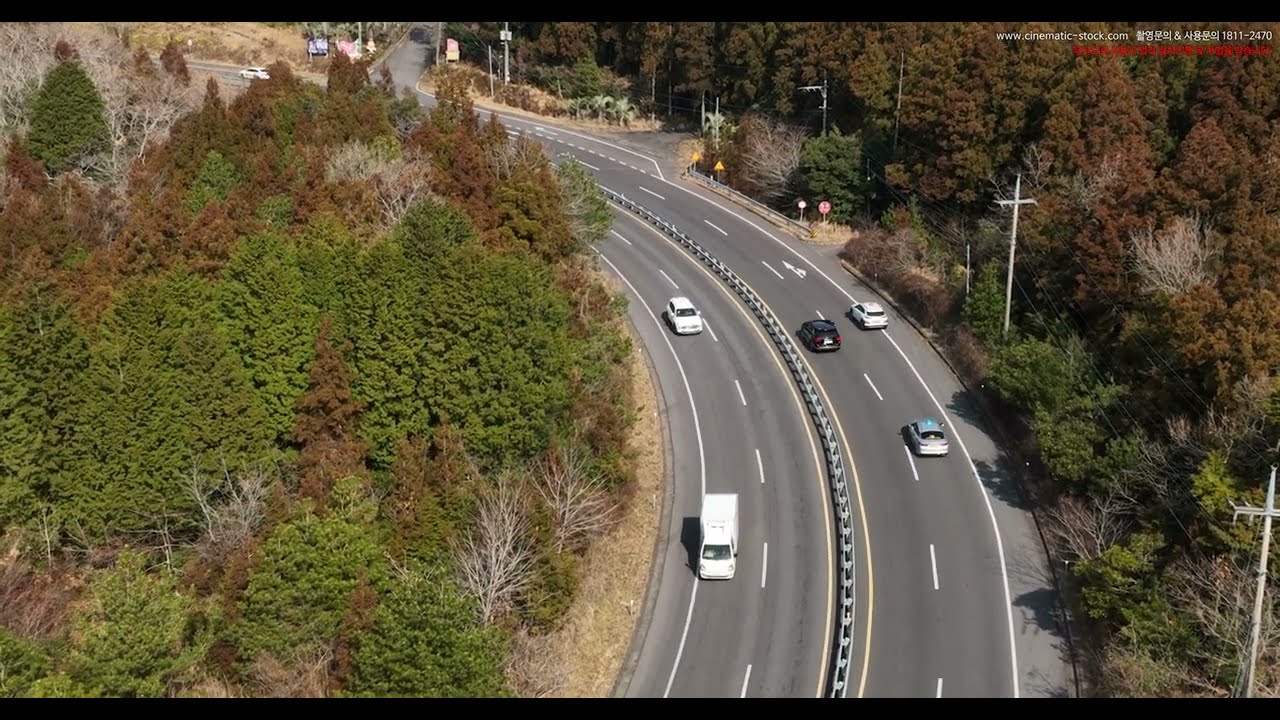The image showcases an overhead view of a dual carriage highway that curves from the center of the image toward the top left. The highway consists of four lanes, two in each direction, divided by a metal median barrier. The road is marked with dashed white lines in the middle and continuous white lines on either side. A white box truck is closest to the bottom of the image, followed by a white car in the same lane. Opposite them, there are several other vehicles, including a black car and another white one. Alongside the roadway, there are utility poles with wires stretching along the right side. The left side of the highway is bordered by a dense forest, primarily filled with trees displaying reddish, orange, and brown hues, but some green foliage is also present. Signage along the road consists of yellow, red, and white signs. The top corner of the image features text: "www.cinematic-stock.com" along with "1811-2470" in white, and some additional Korean text in red. Black strips frame the top and bottom of the image. The overall traffic appears light and flows smoothly, and there’s a noticeable turnoff point at the top of the image leading into another road.